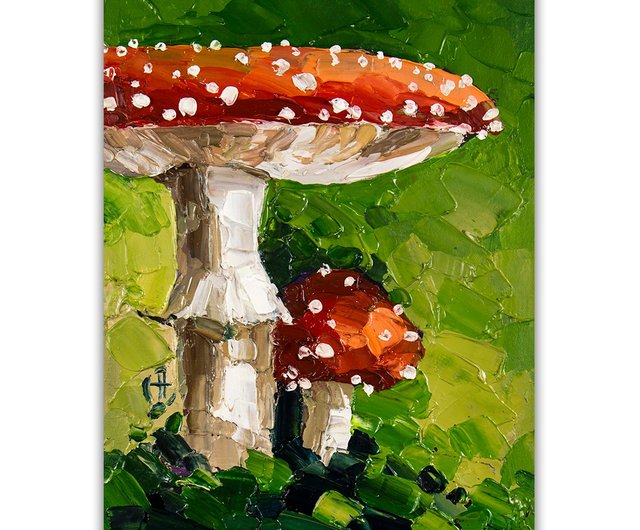This is a detailed oil painting featuring two vibrant red mushrooms, one large and one small. The larger mushroom, characterized by its prominent red cap adorned with white dots, stands confidently towering over the smaller mushroom, which mirrors the same striking cap with white spots. Both mushrooms have white stalks, adding to their distinguished appearance. The painting's background is a rich mosaic of varying shades of green, including dark green, hunter green, and lighter yellow-green, intricately blending to create a sense of depth and grounding. The texture of the paint is palpable, with bold, large strokes and pools of paint contributing to the piece’s tangible, rough surface. The foreground includes nearly black-purple elements, further enriching the painting's complex and layered landscape.